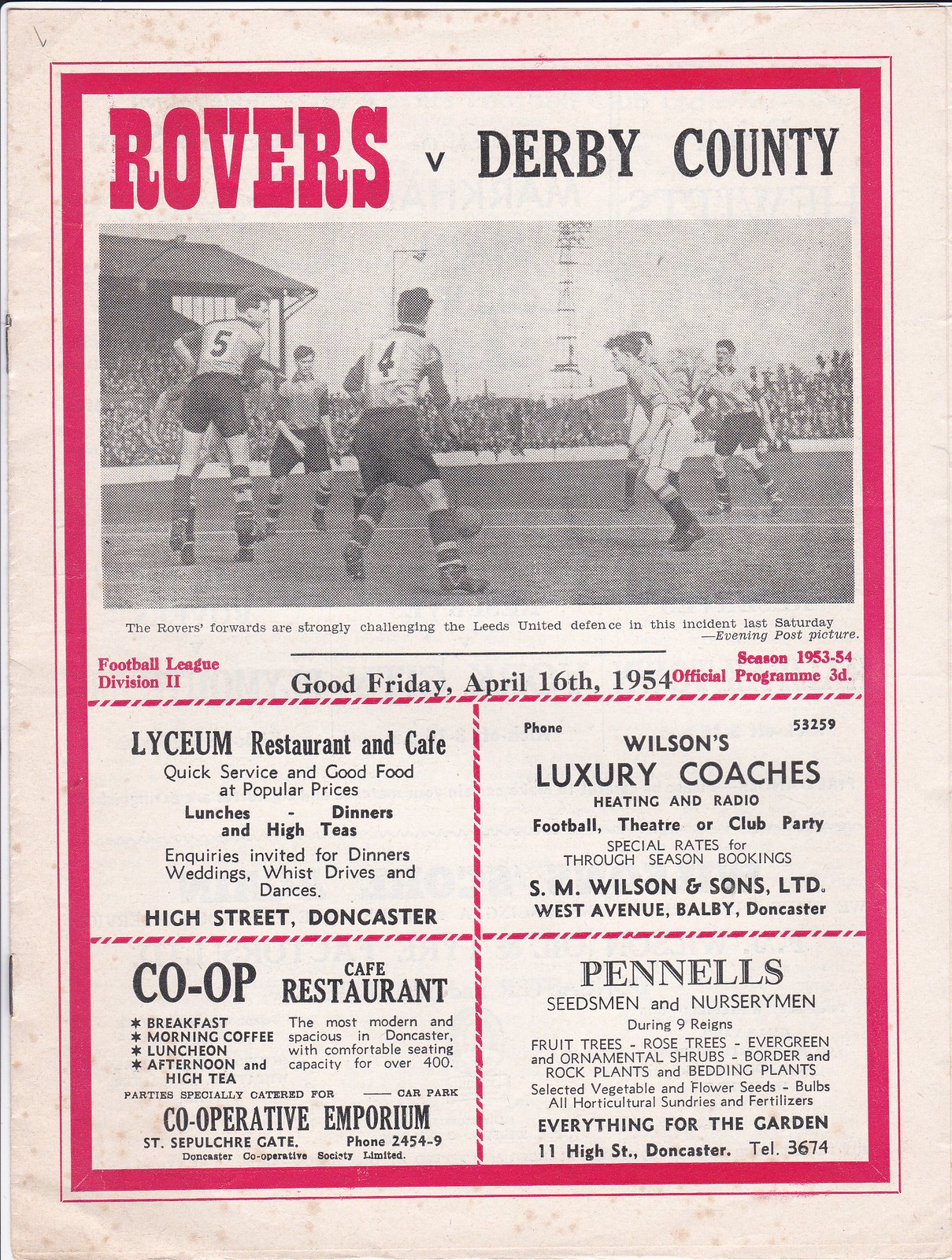The image displays the cover of a vintage sports program for a soccer event featuring a match between the Rovers and Derby County. This aged program cover, on an off-white background with noticeable stains and wear, is framed by a white outer border and a red inner border. The top of the page prominently features the text “Rovers” in red and “v Derby County” in black. 

Centered beneath the text is a black and white photograph of two soccer teams vigorously competing on the field, with a caption underneath stating, “The Rovers forwards are strongly challenging the Leeds United defense in this incident last Saturday evening post picture.”

The lower half of the cover is adorned with multiple advertisements surrounded by striped red and white borders. These advertisers include:

- **Lyceum Restaurant and Cafe**: Offers quick service and good food at popular prices, lunches, dinners, and high teas, located on High Street, Doncaster.
- **Wilson’s Luxury Coaches**: Features heating and radio with special rates for season bookings, located on West Avenue, Holby, Doncaster.
- **Co-Op Cafe & Restaurant**: A modern and spacious establishment, accommodating over 500 guests, offering breakfasts, lunches, teas, and parties, situated at St. Sepulchre Gate, Doncaster.
- **Pennell Seedmen and Nurserymen**: Provides a wide selection of horticultural products including fruit trees, rose trees, and seeds, located at 11 High Street, Doncaster.

This program, dated Good Friday, April 16th, 1954, marks a Football League Division II match for the 1953-54 season, and it was sold for 3d.